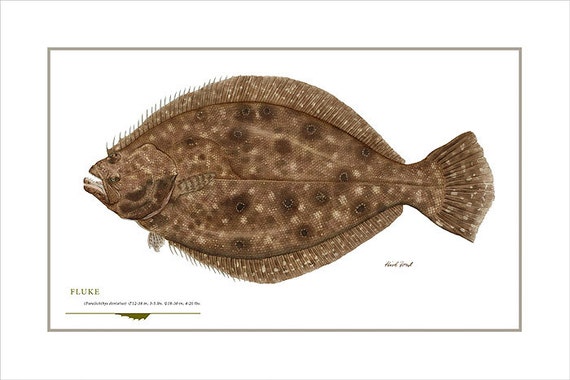This detailed, lifelike illustration captures a fluke—a flat fish, closely resembling a flounder, with both eyes positioned on one side of its face. The fish is depicted swimming on its side, with a body that is tan and adorned with brown spots, each featuring slightly darker central areas. The fluke's elongated dorsal fins stretch from its head to its fan-shaped tail, creating a sense of flow and movement. Its mouth is open, revealing needle-like teeth that give it a predatory appearance. The image, which fits a nature or biology book style, is framed within a white matte bordered by a light brown outline and further enclosed by a thin light gray line, making it perfect for purchase as a print. The fish faces left, accompanied by the label "FLUKE" in uppercase letters at the bottom, adding to the scientific and educational value of the illustration.